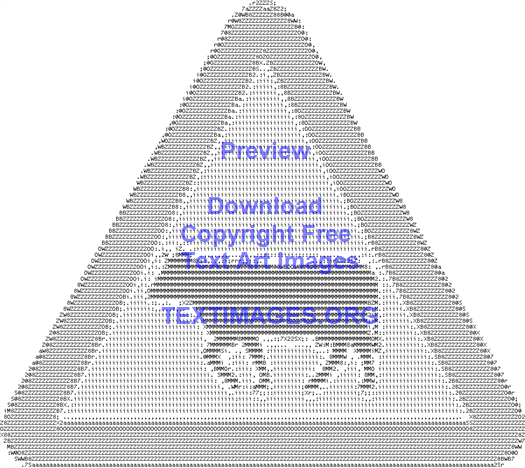The image is a detailed illustration resembling a road warning sign with unique features. It consists of an equilateral triangle with rounded corners, oriented with one point at the top and two at the bottom. The outer triangle is gray with a thick border, and within it lies a smaller, sharper-cornered triangle in light gray. This inner triangle is composed of text characters forming a pixelated texture. Dominating the center of the smaller triangle is a graphic of a cow, rendered in dark gray and appearing to be in motion, lifting its right leg. The image is watermarked with blue text, stating "Preview. Download copyright-free text art images at textimages.org," overlaid in a light lavender purple Arial font. The graphic is visually complex, comprising numerous horizontal lines that may be straining to the eyes. The entire illustration sits on a white background.